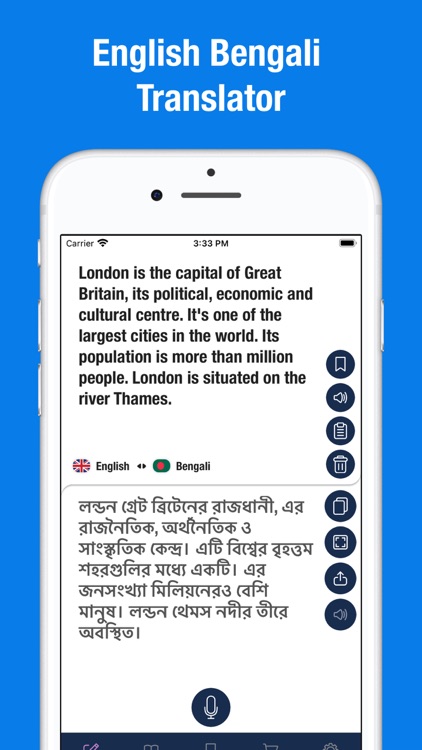Image Description: The image depicts a mobile phone interface showcasing an English to Bengali translation app. At the top, the text "London is the capital of Great Britain, its political, economic, and cultural center. It's one of the largest cities in the world, its population is more than million people. London is situated on the River Thames" is displayed in English. Below this, the translated text appears in Bengali, and just beneath, a microphone icon is visible, suggesting a voice input feature.

On the right-hand side of the screen, a series of icons are arranged vertically, likely representing additional features or tools within the app. The image commentary includes a note of skepticism about London's status as one of the largest cities in the world when compared to cities like Phoenix, Arizona.